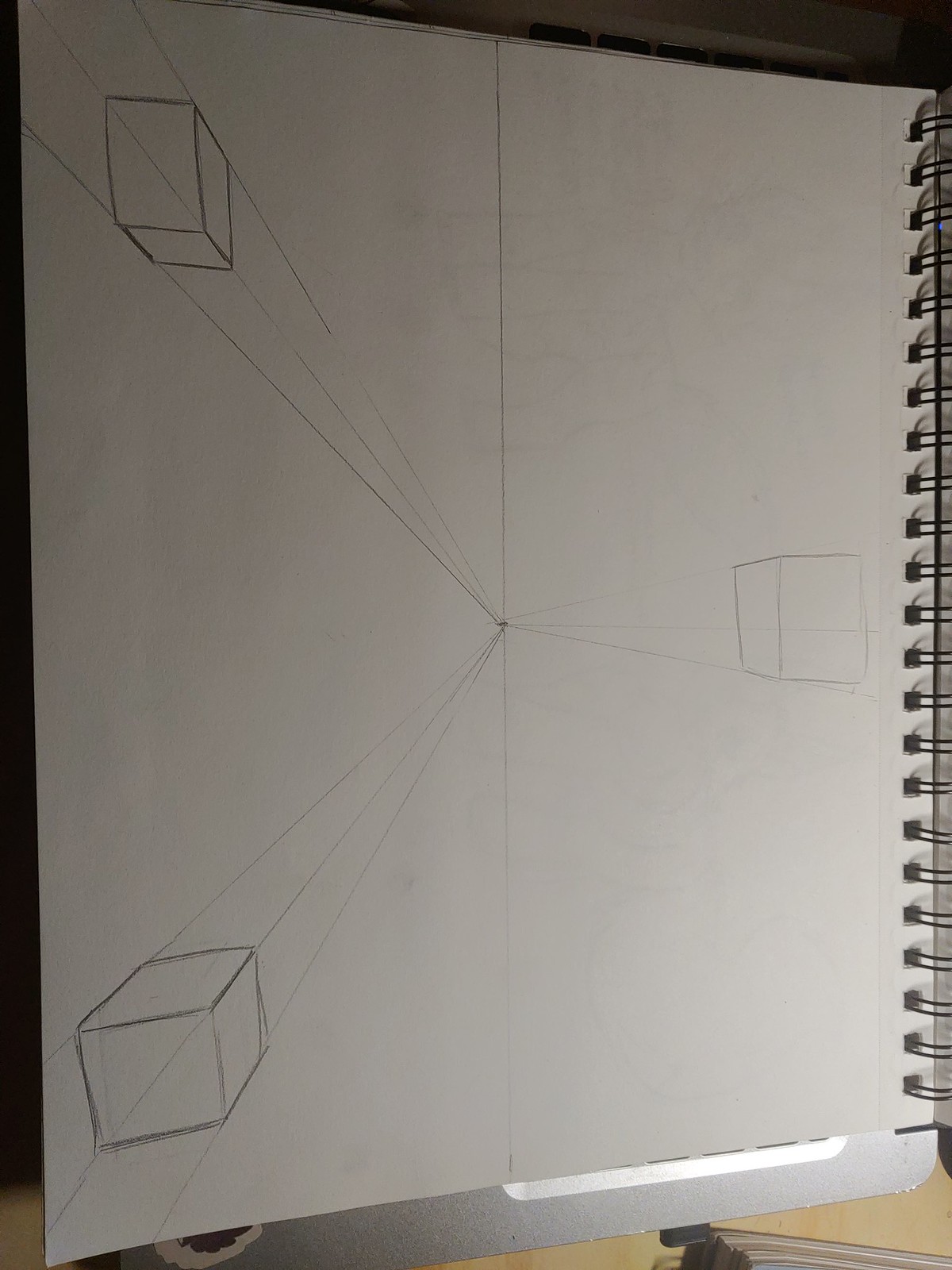The image depicts a spiral notebook viewed from above, with the spiral binding prominently displayed along the far right edge, running vertically down the page. The metal clasps of the spiral binding are clearly visible, securing the pages together. On the notebook page, three rectangular boxes have been sketched, each rendered with lines to create a three-dimensional effect. The first box is positioned at the top left, the second at the bottom left, and the third in the middle right of the page. 

Faint diagonal stripes are drawn within each box, and these stripes converge at a single point in the center of the page, creating a sense of perspective and unity among the boxes. Additionally, a vertical line intersects the page, passing through the central convergence point of the diagonal stripes. 

Beneath the notebook, a contrast of colors is visible: a light gray surface transitions into a darker gray, suggesting the presence of a second object, possibly another piece of paper or a clipboard. To the right of this darker gray surface, a small piece of white paper is noticeable. The backdrop features a beige surface that likely represents a table. Partially obscured and situated below these layers, the barely discernible top of a pair of glasses can be seen.